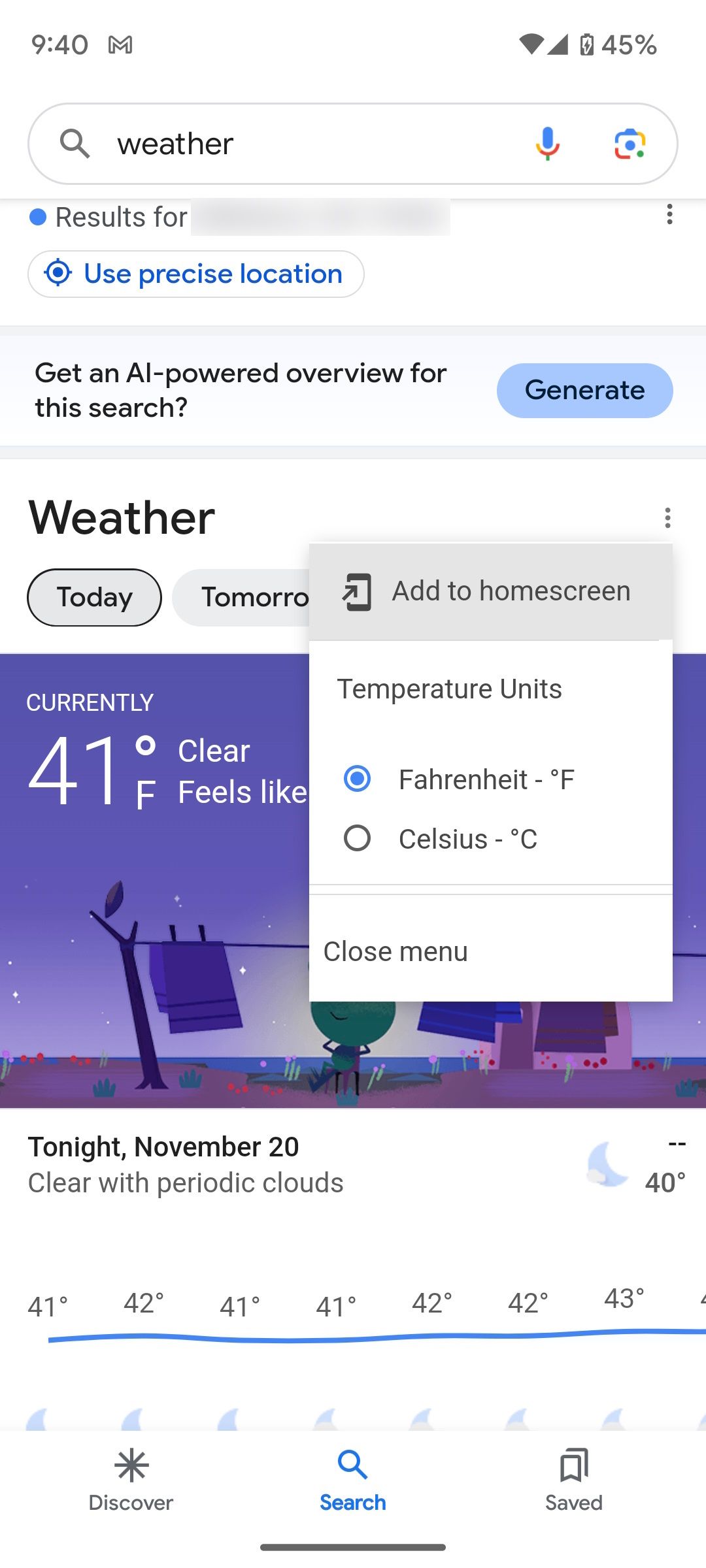Here's a detailed, cleaned-up descriptive caption for the image:

---

A screenshot displays the current weather information on a mobile device. The time on the device shows 9:40 AM, with the battery life at 45%. The user has conducted a Google search for weather which utilizes precise location data. The search interface prompts the user with options including "Add to Home Screen" and settings for "Temperature Units" (Fahrenheit or Celsius). These options are partially obscured by an open menu.

The current weather report indicates that it is a clear day with a temperature of 41 degrees Fahrenheit. The "Feels Like" temperature is not visible. The background image features a picturesque scene of a clothesline with various garments hanging to dry. 

For the evening of November 20th, the forecast predicts clear skies with occasional clouds and a consistent temperature pattern ranging from 40 to 43 degrees Fahrenheit. The hourly temperature progression is detailed as 41, 42, 41, 41, 42, 42, and then 43 degrees Fahrenheit. 

At the bottom of the screenshot, options such as "Discover," "Search," and "Saved" are available for further navigation.

---